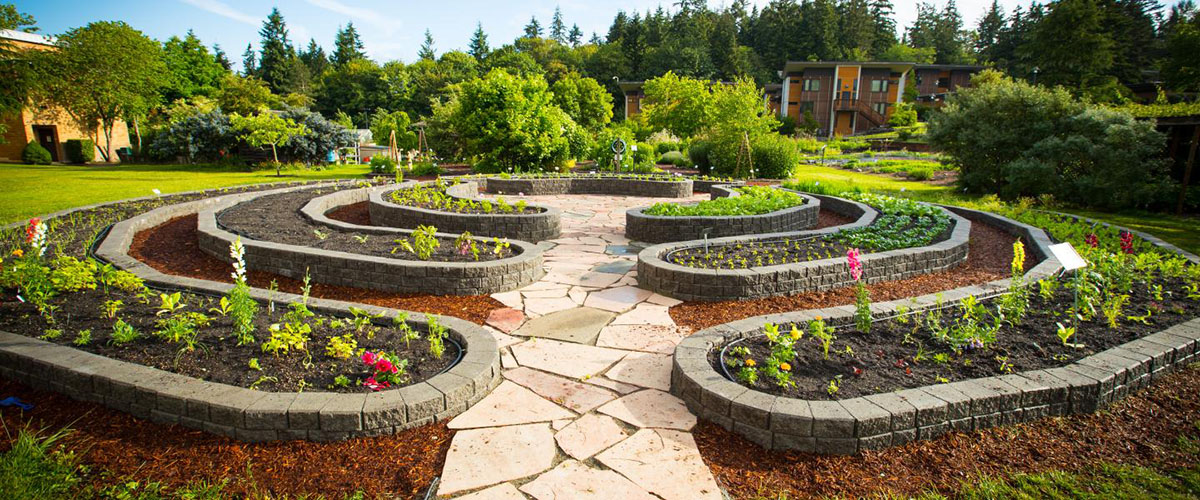The image depicts a newly constructed garden, possibly situated in an apartment complex or a small college campus, featuring a meticulously designed layout with raised concrete beds forming concentric circles. The garden is divided into three almost-complete circular sections, with walkways made of light tan, irregularly-shaped stones—triangular, square, and random forms—connecting them. The largest outer circle seems to be densely planted with a variety of flowers and small shrubs, displaying a vivid array of colors at this early stage of growth. The beds are constructed with cement-gray colored walls that are fairly shallow. In the middle of the arrangement, there is a patio area, adding a communal touch to the space. Overhead, the sky is a light turquoise blue, while the background is framed by tall, dark green evergreen trees, enhancing the serene and picturesque ambiance of the garden.